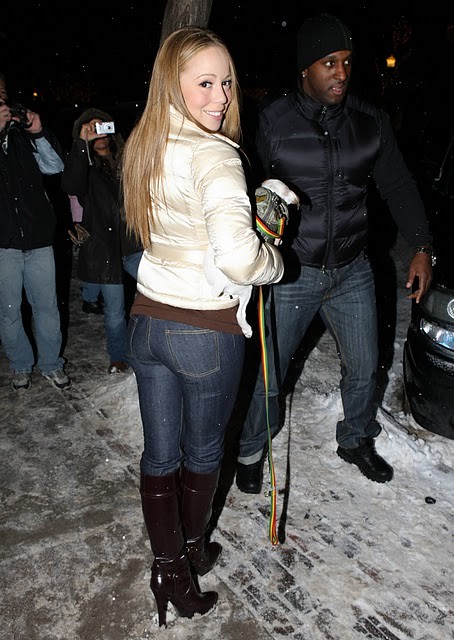The photograph captures singer Mariah Carey standing at the center of the scene against a snowy, nighttime backdrop. Mariah has straightened blond hair and light skin, adding a touch of glamour with a stylish cream-colored puffer jacket over a brown shirt. She pairs this ensemble with jeans and high-heeled black boots. In her arms, she holds a small white puppy adorned in a colorful coat and clutching what appears to be a rainbow-colored leash. Mariah is looking back directly at the camera, her head tilted to create engaging eye contact.

In the foreground, the snowy ground is partially visible, with snow piled up around what seems to be a sidewalk. A dark tree trunk stands right in front of Mariah, adding an element of nature to the urban setting. To the left and somewhat in the background, there are several people snapping pictures of her, capturing the moment. 

To her right stands a man, likely African-American with dark skin, dressed in a black beanie, black jacket, and jeans, who appears either as a bodyguard or a close acquaintance. He is positioned closer to Mariah, unlike the other photographers who maintain a respectful distance. Additionally, the front end of a dark-colored car, possibly dark blue or black, is barely visible, cropped at the right edge, with its headlights pointing towards the scene. The overall atmosphere is accentuated by the nighttime darkness, emphasizing the black background that frames the image.